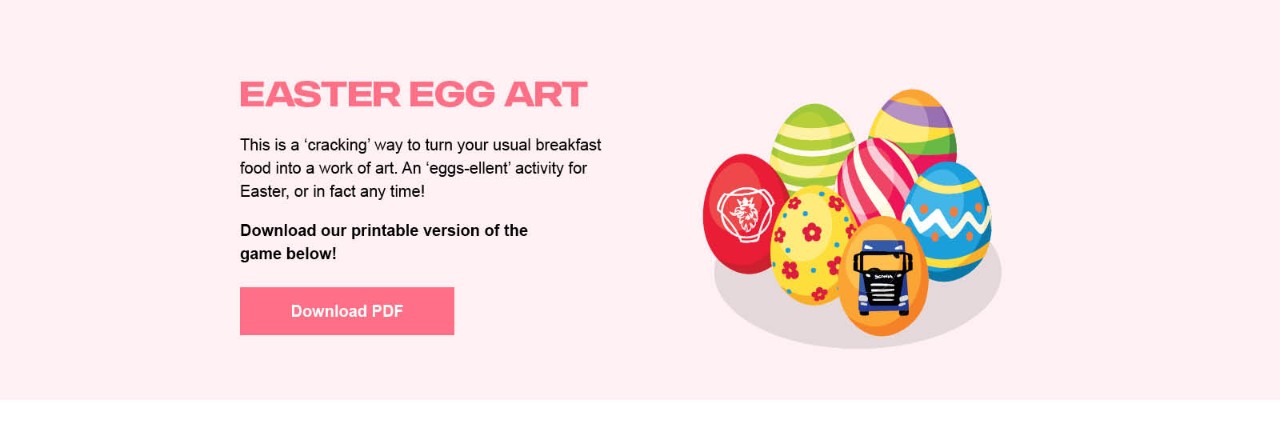The image titled "Easter Egg Art" features a computer-generated display of seven intricately designed Easter eggs arranged in a semi-circle against a beige background. The entire scene is set against a pink backdrop, adding a festive and vibrant touch. The title "Easter Egg Art" is prominently displayed at the top in capital letters, rendered in a darker pink shade for emphasis.

Beneath the title, there is a playful description that reads, "This is a ‘cracking’ way to turn your usual breakfast food into a work of art." Following this, another phrase highlights the activity as an "egg-cellent" (with "eggs" capitalized for a pun effect) activity suitable for Easter or anytime, punctuated by an exclamation point.

In bold print, there’s a call to action that states, "Download our printable version of the game below." Directly beneath this text is a clickable rectangle button labeled "DOWNLOAD PDF," with "PDF" in capital letters.

The seven Easter eggs each boast unique and colorful designs. One egg features an image of a semi-truck, while another showcases red flowers on a yellow background. There is an egg adorned with a pattern of green, yellow, and white stripes. Among the collection is a solid red egg, a multicolored striped egg, and another with teal, white, and yellow stripes accompanied by orange dots.

This detailed presentation not only highlights the artistic aspect of Easter eggs but also invites viewers to engage with the content by downloading and participating in the activity.